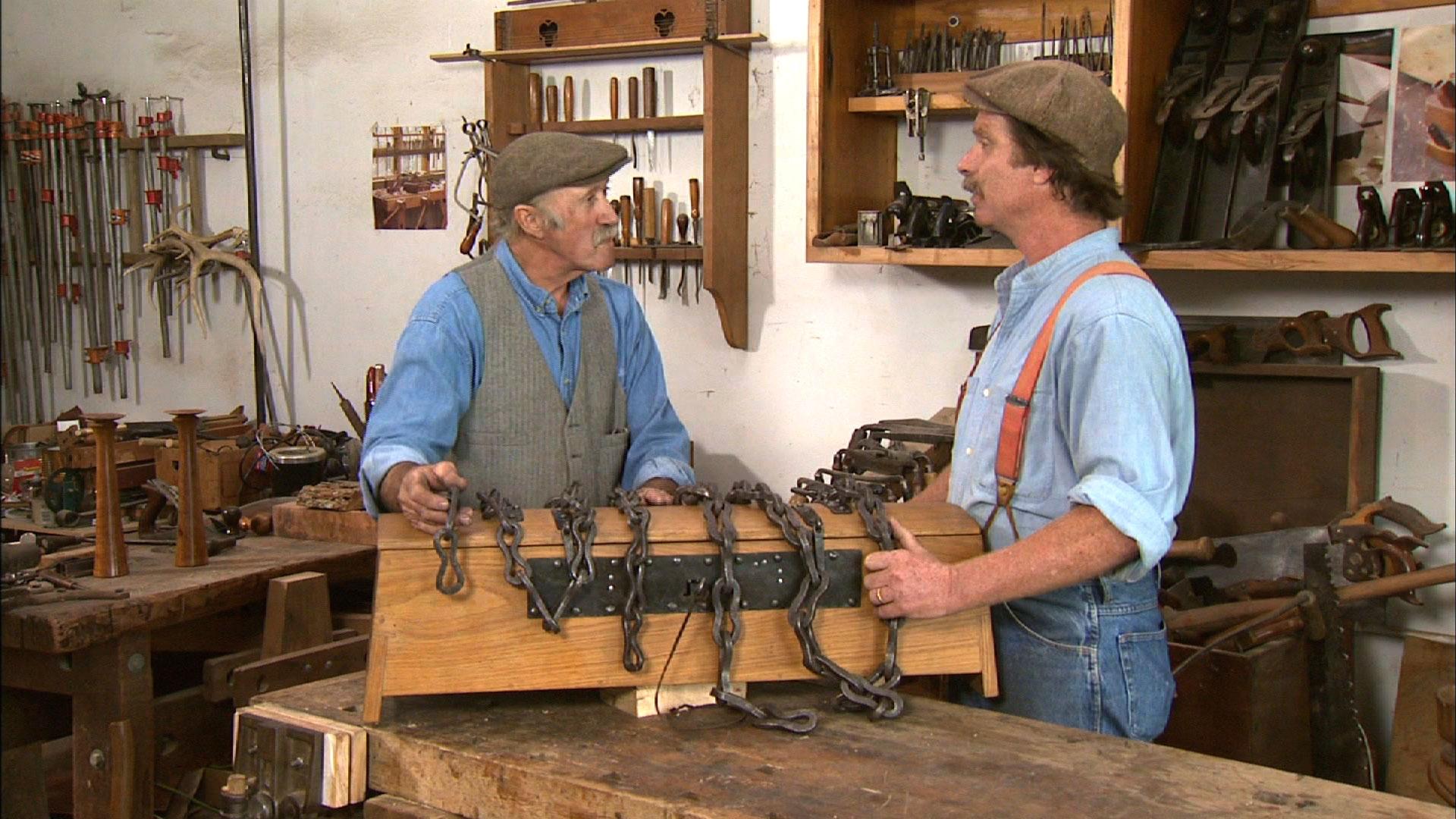In the bustling ambiance of a woodworking shop, two men stand across from each other, engaged in a focused conversation. To the left of the image is an older gentleman with a hint of a gray mustache, wearing a flat brown hat, a blue denim shirt with sleeves rolled up, and a buttoned-up gray vest. His body turns slightly to the right as he leans over a long wooden workbench. Opposite him, to the right, stands a younger man sporting a brown cap and curly brown hair, with a light blue button-up shirt and bright orange suspenders over blue jeans. His left hand reaches over chains that crisscross a large wooden box on the bench. Both men grasp the chains, contemplating their next move. The workshop walls behind them are lined with various tools, including hand saws and carving implements, neatly arranged in racks. To the left, an additional work table cluttered with objects hints at ongoing projects. The detailed setup underscores the meticulous craftsmanship inherent to the space, drawing viewers into the intimate world of these skilled artisans.